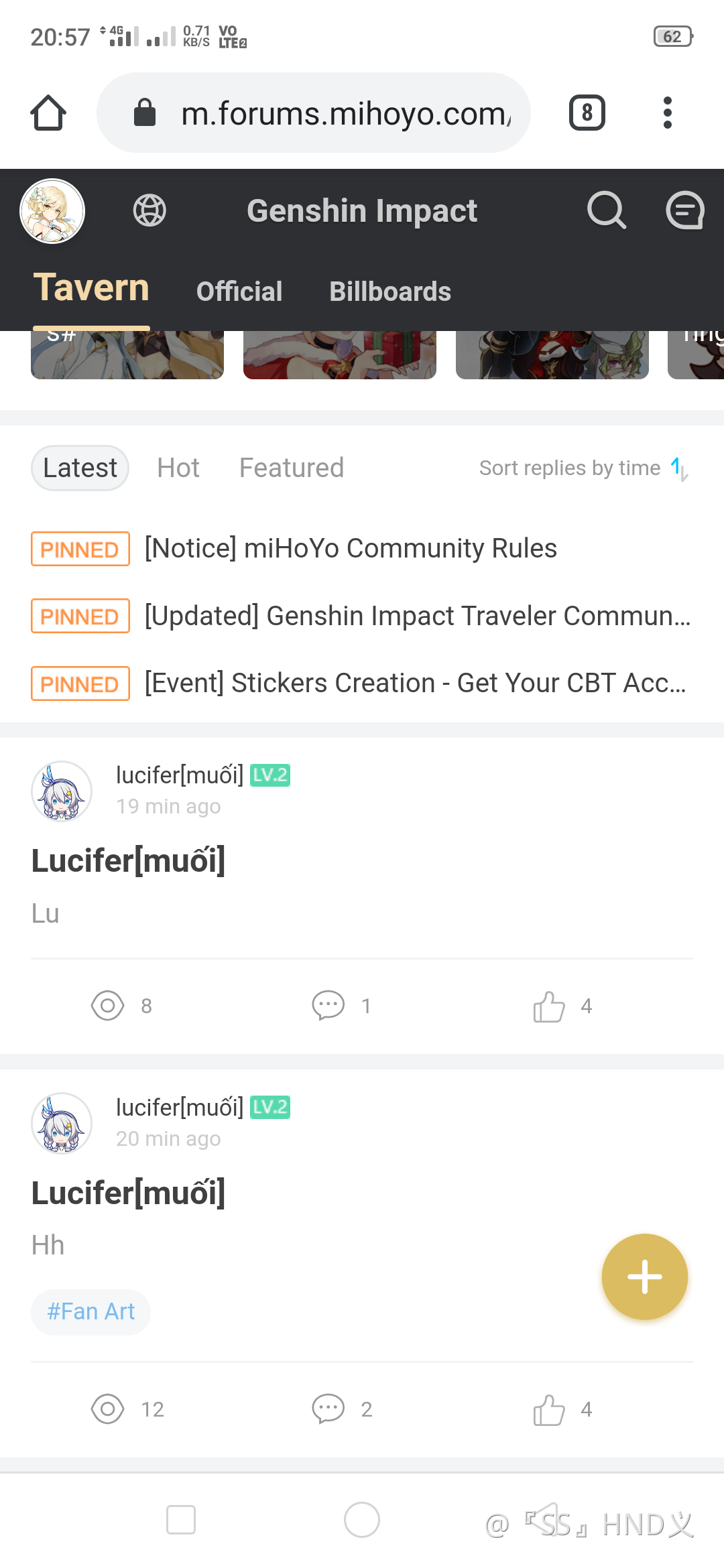This is a screenshot captured from a cell phone displaying the website m.forums.myhoyo.com. At the top of the screen, a dark gray rectangle prominently features the title "Genshin Impact." The user has selected the "Tavern" section from the menu, which also includes options like "Official" and "Billboards." The Tavern area shows a series of pinned posts, all highlighted in orange rectangles. These posts include "Notice: Myhoyo Community Rules," "Genshin Impact Traveler Communicate," "Event Stickers," "Creston Creation," and "Get Your CBT Account." Below these pinned posts, the username "Lucifer Mui" appears twice. In the lower-right corner of the screen, there is a mustard yellow circle with a white plus sign inside it.